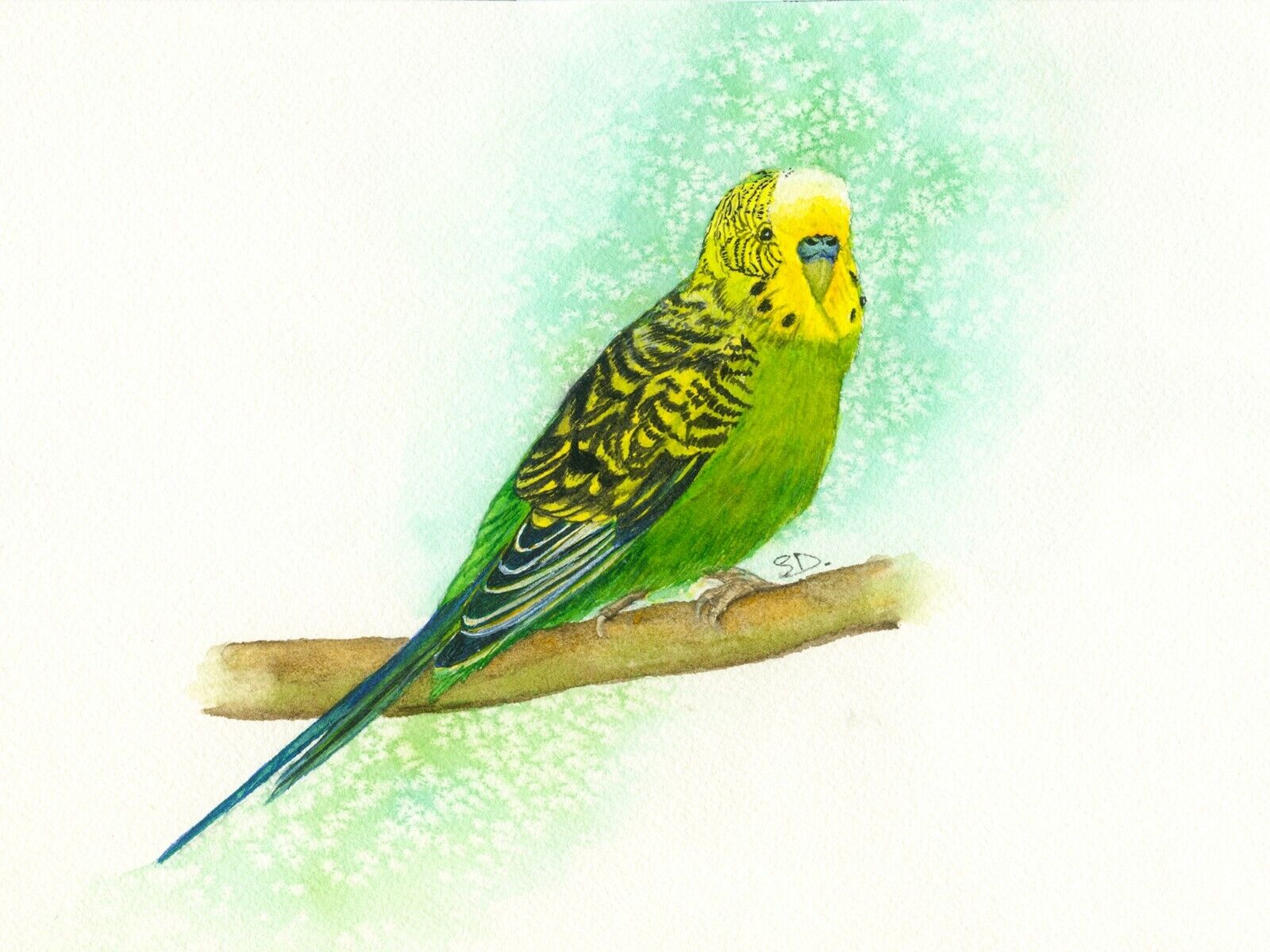This is a meticulously detailed watercolor painting of a vibrant parakeet perched on a light brown, slightly upward-sloping branch. The parakeet, facing left, showcases a brilliant palette of colors: the face is adorned with bright yellow feathers interspersed with black lines, highlighting small black eyes. The beak, almost flat against its face, is light green with a touch of blue where the nose would be. The bird's chest transitions from hypnotic lime green down to teal, continuing in this vibrant green that peaks through its tail feathers. The bird's wings, awash with yellow and black feathery patterns, contrast sharply against its green breast. As one visually traces the bird towards its tail, the feathers end in a rounded, black form with white stripes, transitioning to a long, pointed feather that concludes in a captivating blue hue.

The background of the painting subtly enhances the bird's vivid colors, with a light green hue dappled with white speckles in the upper right, gradually fading to white near the edges. The overall simplicity of the background keeps the focus firmly on the parakeet. The lower part of the image, near where the bird perches, features a signature in French, "BD," confirming the artist's touch. This parakeet illustration encapsulates a delightful blend of detailed artistry and brilliant splashes of color, resonating with the simplicity and elegance of watercolor techniques.